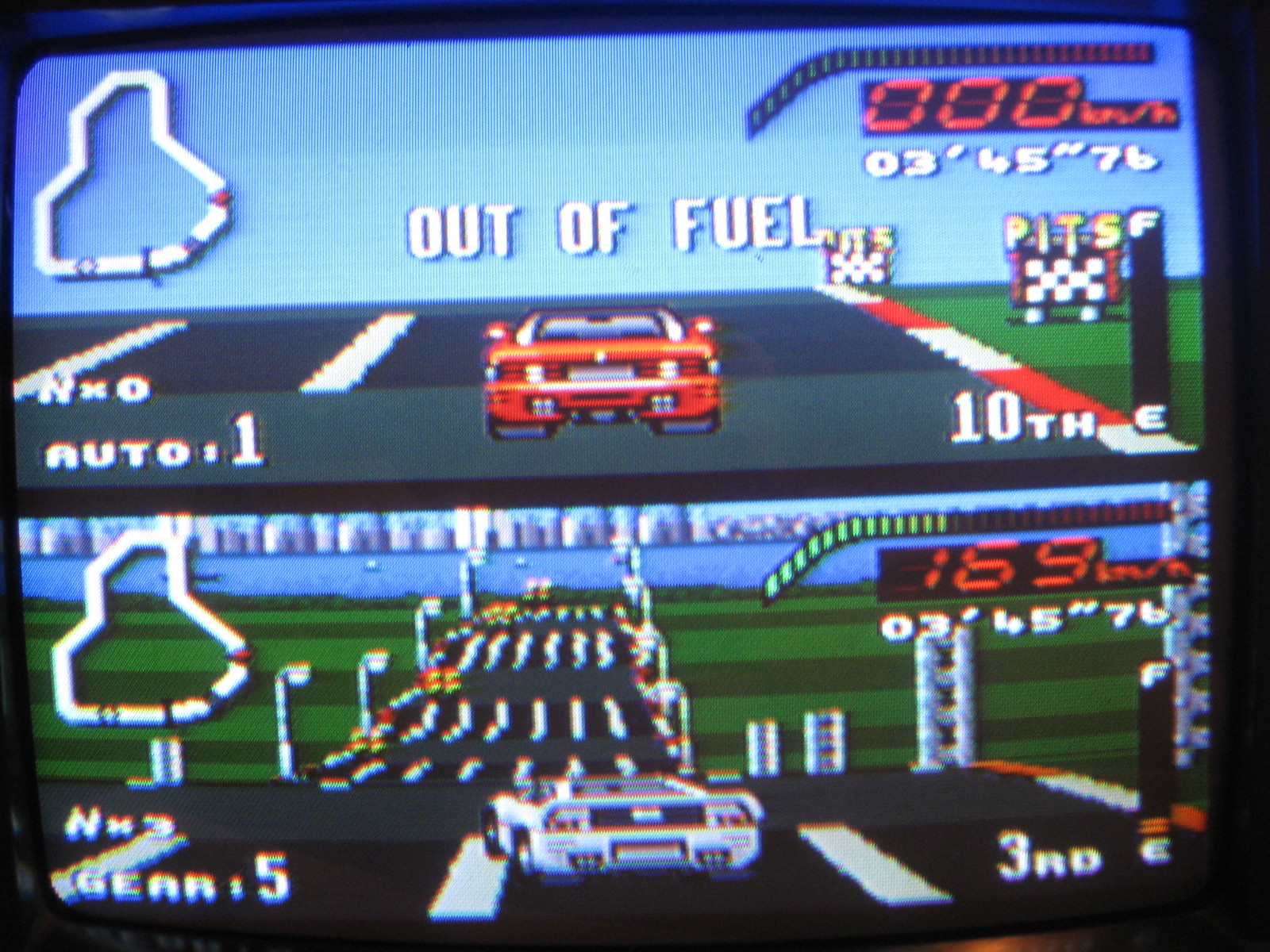This image captures a nostalgic moment from an early video game, presenting a split-screen view of a racing scenario. The upper half of the screen features a red car on a racetrack, accompanied by a bold message in white capital letters stating "OUT OF FUEL." To the right of the red car, a black pole with a black and white checkered sign marked "PITS" signifies the pit stop area. In the top right corner, the player is shown in 10th place with a speedometer reading zero miles per hour. To the left, a simplified white map of the racetrack is displayed.

In the lower half, a white car races ahead, currently holding 3rd place, speeding at an impressive 169 miles per hour. The road extends into the distance, adorned with light posts on either side, each bearing a lit lamp, creating a classic race day atmosphere. This snapshot captures the essence of vintage gaming, merging competition and the era's vivid graphical storytelling.